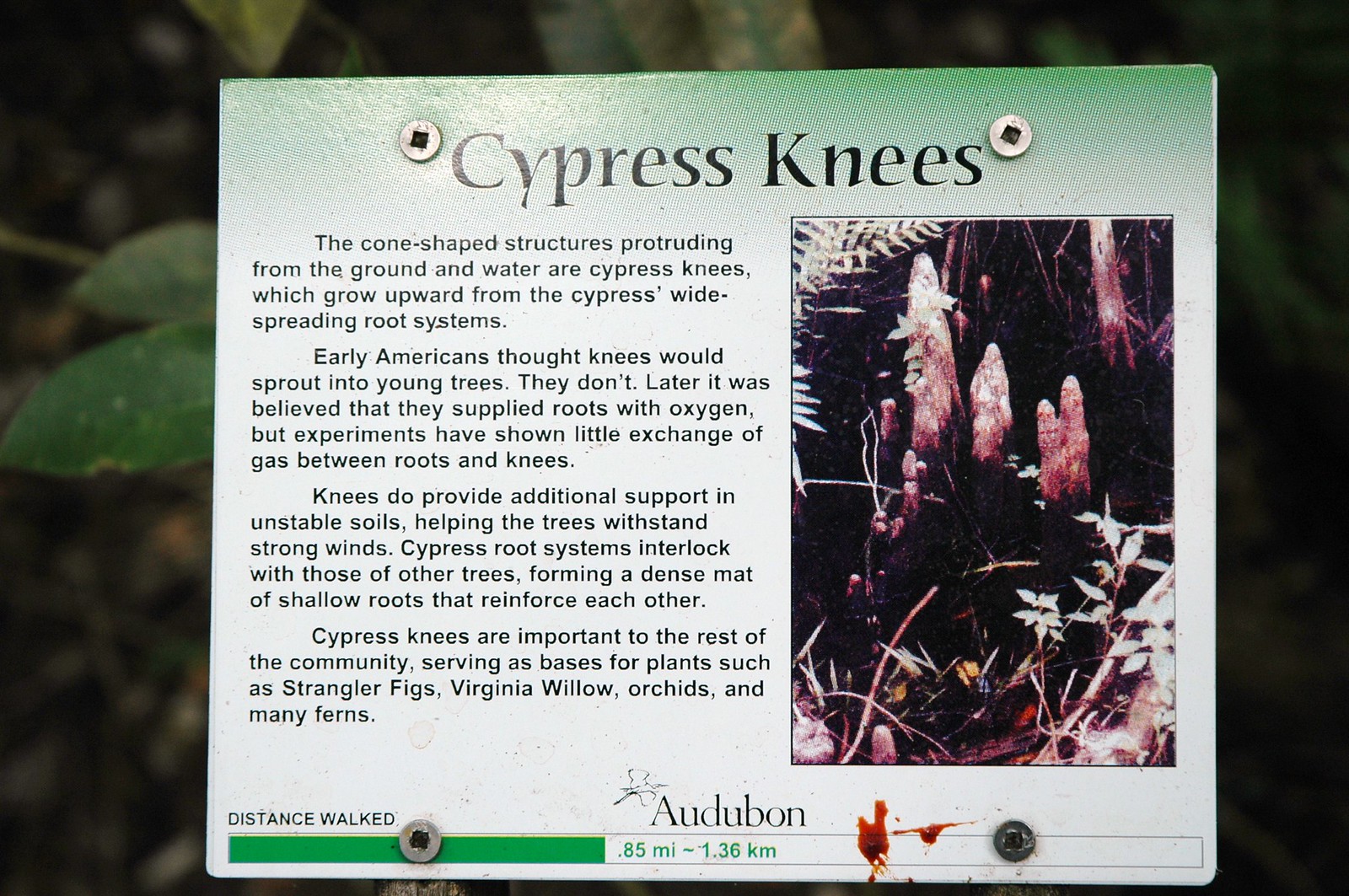This image is a detailed, close-up photograph of an outdoor informational sign centered prominently in a natural setting. The sign is titled "Cypress Knees" and is primarily made of metal, secured with four visible metal screws at the top and bottom. The left side of the sign features descriptive black text on a pale background, detailing the unique features of cypress knees – cone-shaped structures that grow from the widespread root systems of cypress trees. The text explains their misconception as potential new trees, their debated role in providing oxygen to roots, and their actual function in stabilizing trees in unstable soils. Moreover, these structural roots support a community of other plants, such as strangler figs, Virginia willow, orchids, and many ferns.

On the right side of the sign, there is a large photo, slightly blurry, depicting the cypress knees. Below the text and image, there is a green progress bar indicating "Distance Walked: 0.85 miles (1.36 kilometers)," suggesting that the sign is part of a wildlife trail, sponsored by Audubon. The background of the photo shows indistinct greenery, including plants and trees, adding to the natural context of the setting. A small red blood stain near the bottom right screw suggests a minor injury occurred, possibly from someone grazing their hand against the sign.